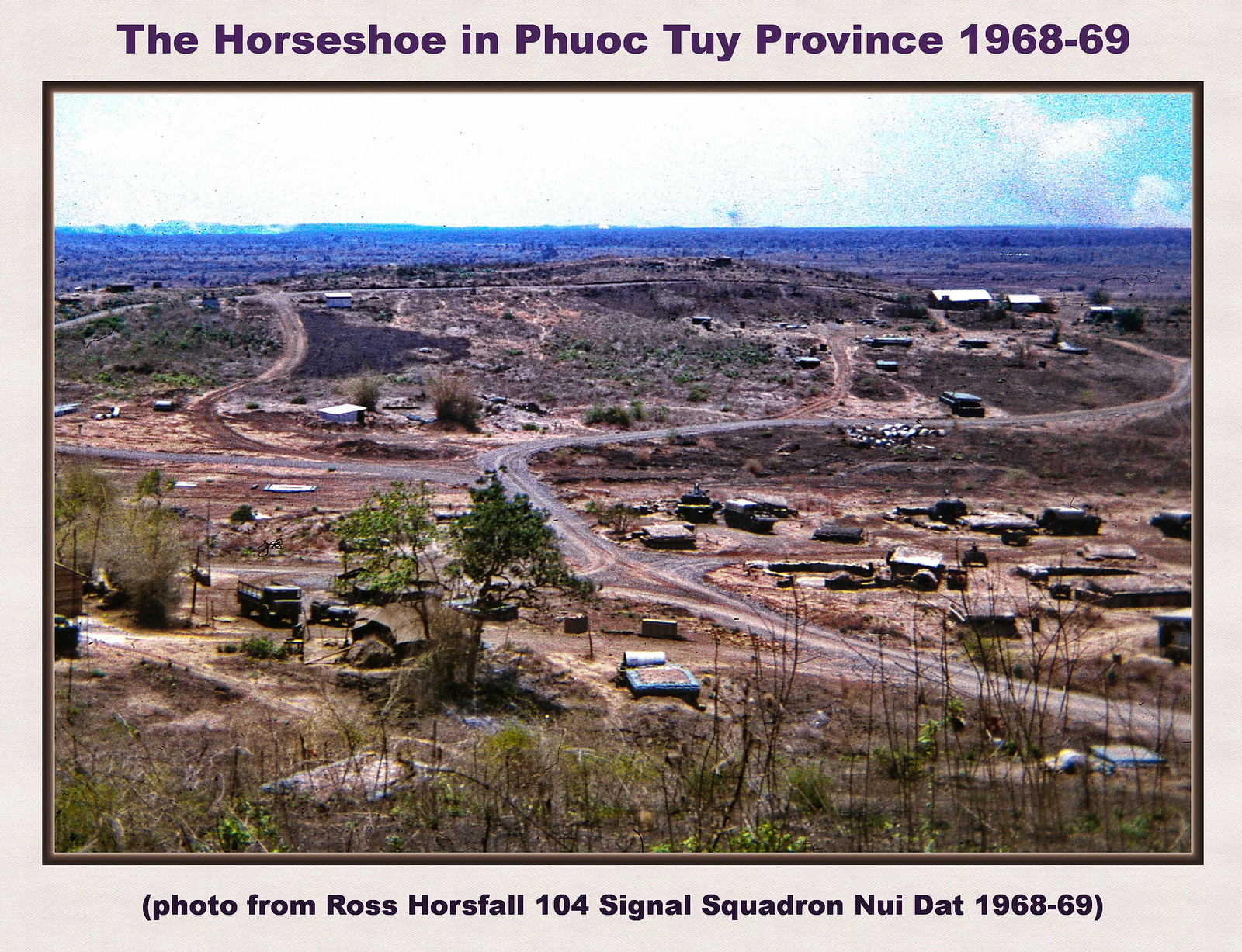This image, bordered in gray, depicts an aerial view of The Horseshoe in Phuoc Tuy Province from 1968-69, with credit given to Ross Horsfall from the 104 Signal Squadron, Nui Dat, for the photo. The photograph, with a faded, vintage quality, shows a sparsely populated town during the daytime under a mostly cloudy sky with patches of blue. In the foreground, there are patches of dry grass and scrub, accompanied by a few vehicles and sparse trees. The town features a small hill with several building structures, including houses and a few other buildings scattered around. A dump truck with dirt is also visible. Roads connect different parts of the town, although the overall infrastructure appears minimal. The horizon and distant elements such as hills or mountains can be seen in the background, enhancing the sense of depth in the image.